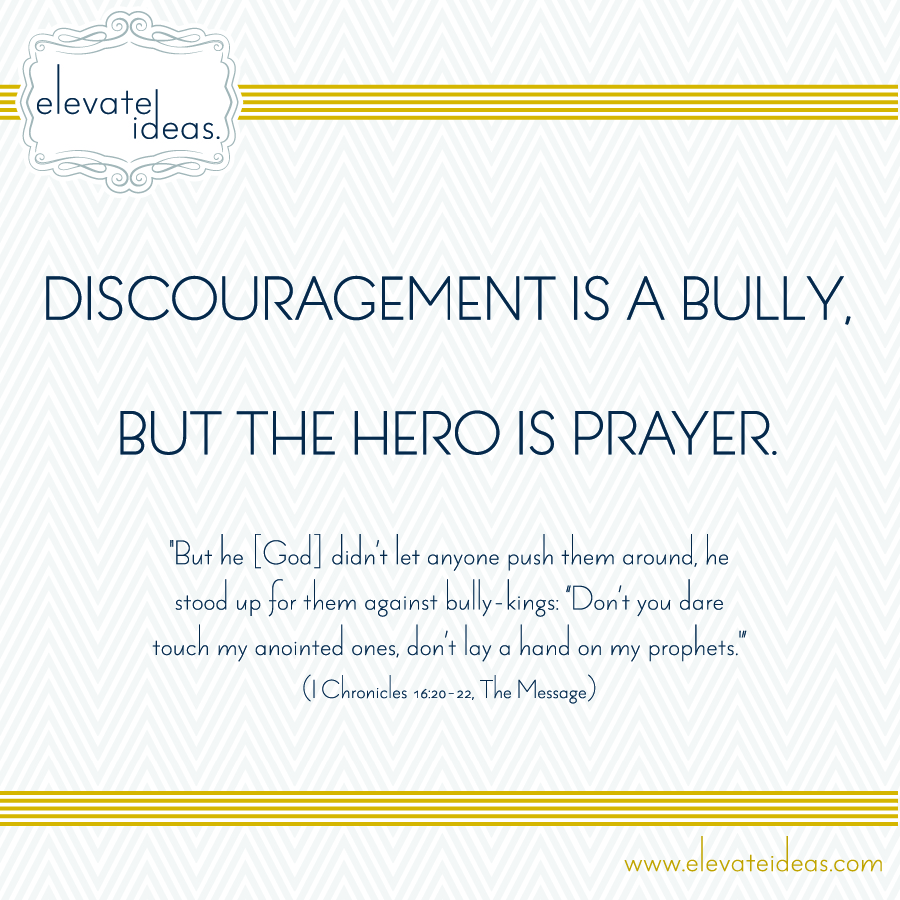The image features an inspirational quote, typical of those seen on Instagram, with the main quote in all caps blue text reading: "DISCOURAGEMENT IS A BULLY, BUT THE HERO IS PRAYER." Directly underneath, in smaller text, is a Bible verse from 1 Chronicles 16:20-22 (The Message): "But he, God, didn't let anyone push them around. He stood up for them against bully kings. Don't you dare touch my anointed ones. Don't lay a hand on my prophets." 

This quote graphic is set against a white background adorned with a frilly ornamental border and a busy, gray and white triangular, wavy pattern. At the top and bottom of the image, there are horizontal gold bars running from left to right, each consisting of five narrow bars with white spaces in between. The upper left corner features a logo or badge that reads "Elevate Ideas" surrounded by scrolling artwork. In the lower right corner, the website, www.elevateideas.com, is printed in gold.